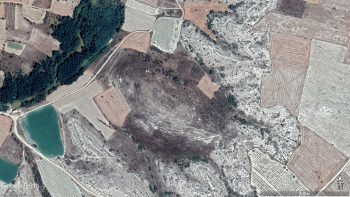This aerial photograph offers a detailed top-down view of a land area that includes various features like buildings, ruins, and an excavation site. The landscape appears to be divided into different plots and fields, some rectangular in shape and delineated by straight lines indicative of human planning. Centrally, there is a large, circular excavation site, with gray sand or soil oozing around its perimeter. Some buildings sport red rectangular roofs, while others have gray rooftops. Towards the upper left, a patch of dense green trees contrasts with the otherwise sparse terrain. The bottom left portion features a road running through it, flanked by greenish-blue bodies of water that resemble small ponds or a swimming pool-like structure. Overall, the setting appears undeveloped and stylistically designed as an excavation site.